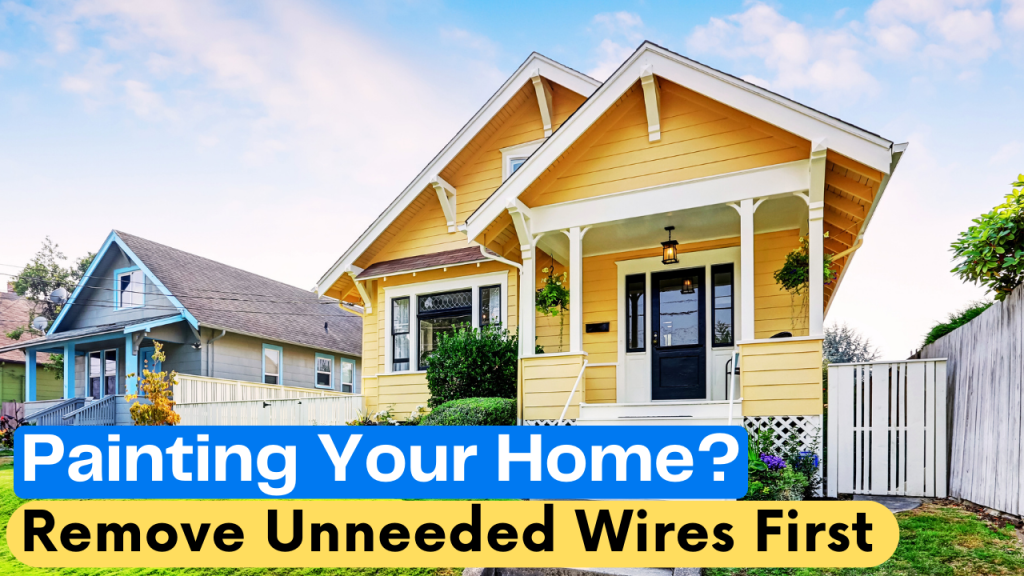The image is a detailed photograph, possibly an advertisement or public service announcement, centered around a prominent yellow house. This wooden house is painted yellow with white trim and has horizontal planks. A small front porch with white steps and a black door featuring a glass section near the top is visible, along with a white latticework covering a crawl space or basement area underneath. Off to the left, there is another long, one-story house with a predominately gray color accented by light blue trim. In front of the yellow house, there's a green, grassy yard bordered by a white fence on the right, leading to a side door. Above the black door of the yellow house, a lamp is hanging. The bottom section of the image contains text: In a rounded blue rectangle with white letters, it reads "Painting your home?" Beneath that, in a yellow strip with black letters, the text advises, "Remove unneeded wires first."